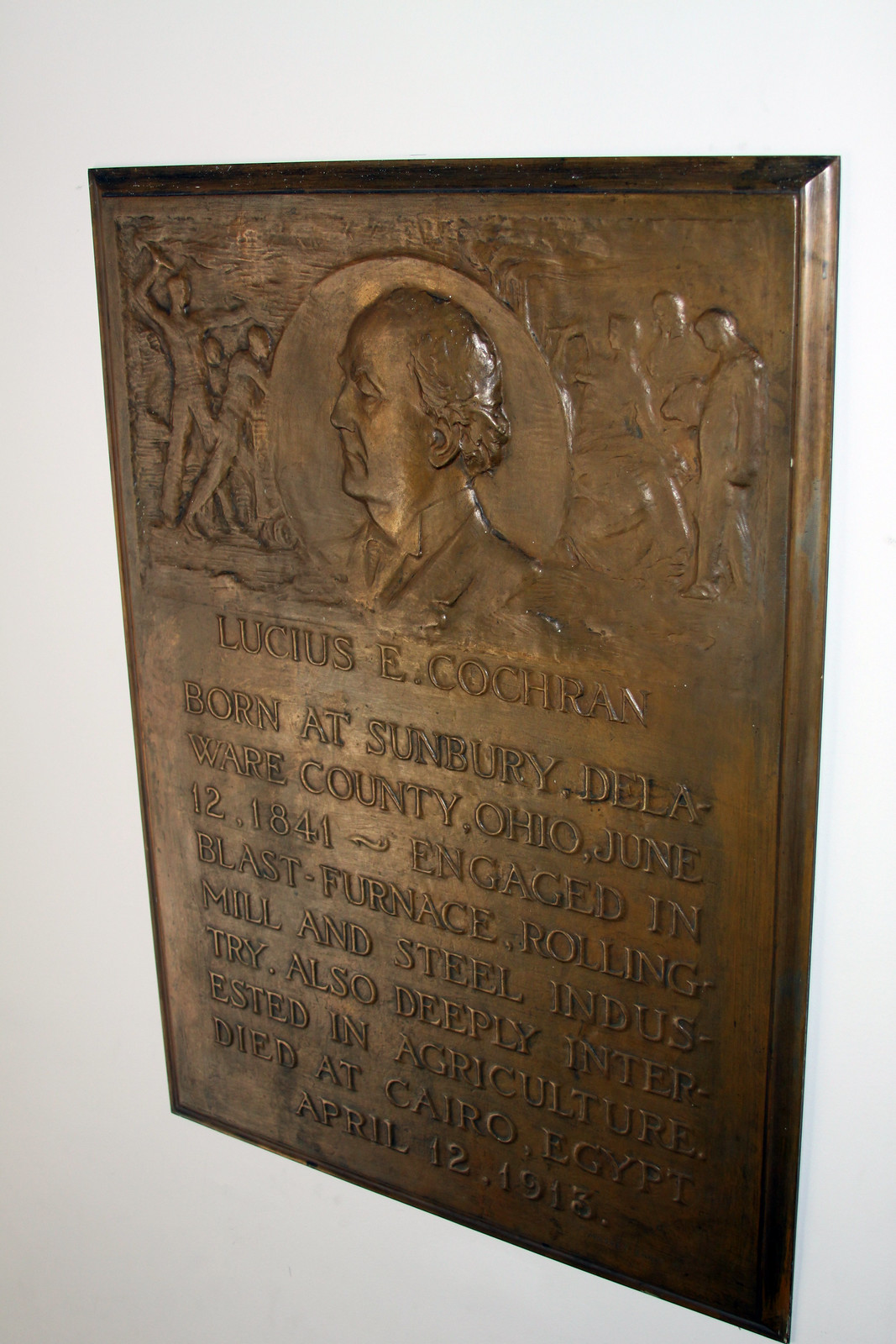The image features a bronze placard, securely attached to a white wall and photographed at an angle that makes the right side appear larger due to perspective. The top section of the placard showcases intricate carvings depicting people engaged in industrial work, along with a central portrait medallion of Lucius E. Cochran. The detailed bust portrays Cochran as an older man with a receding hairline, prominent forehead, and medium-length hair. He is dressed in a collared shirt. Below the artwork, the raised text reads: 

"Lucius E. Cochran, born at Sunbury, Delaware County, Ohio, June 12, 1841. Engaged in blast furnace, rolling mill, and steel industry. Also deeply interested in agriculture. Died at Cairo, Egypt, April 12, 1913."

The bronze material is distinguished by its embossed (rather than engraved) text and imagery, adding a tactile richness to the historical commemoration.